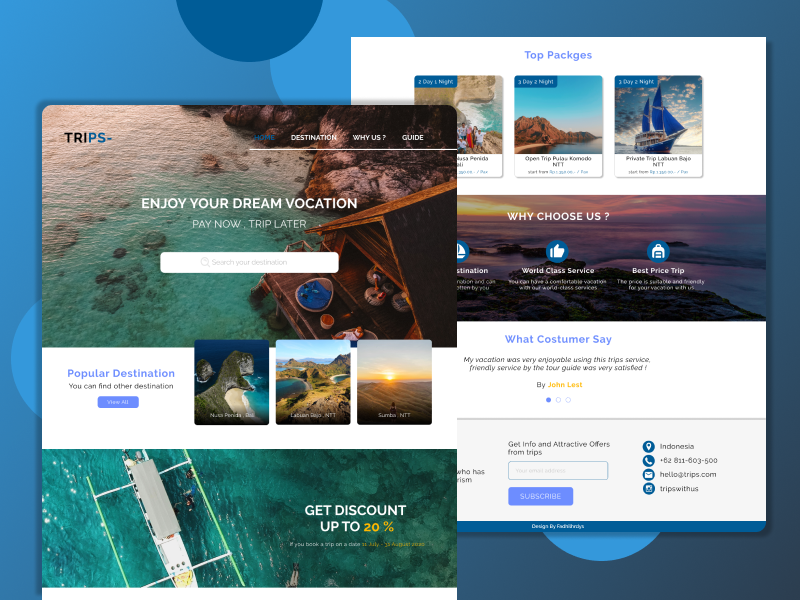The image depicts two separate web pages with contrasting blue backgrounds. The left side features a lighter blue background adorned with three partially visible light blue circles and a dark blue circle. 

The first web page on the left is titled "Trips" using a mix of black and blue letters. It categorizes options into three sections, all highlighted in white: "Enjoy a dream vacation," "Plan your trip later," and a search bar. Below this, the text reads "Popular Destination," accompanied by a blue button and three enticing images of vacation spots. Further down, there's a section offering discounts up to 20%, featuring an image of a turquoise blue-green ocean and a yacht. The topmost image is of a brown cabin seemingly floating on water.

The second screen, set against a darker blue background on the right, begins with the header "Top Packages" in blue. Directly below this, three travel packages are displayed. A section titled "Why Choose Us" follows, set against a sunset over water backdrop, detailing three service features: "World-Class Service" (center), "Best Price Trips" (right), and one partially obscured option (left). Below this, customer reviews are introduced with the subheading "What Customers Say" in blue text. At the very bottom, there is a subscription section where users can input their information, capped by a blue footer.